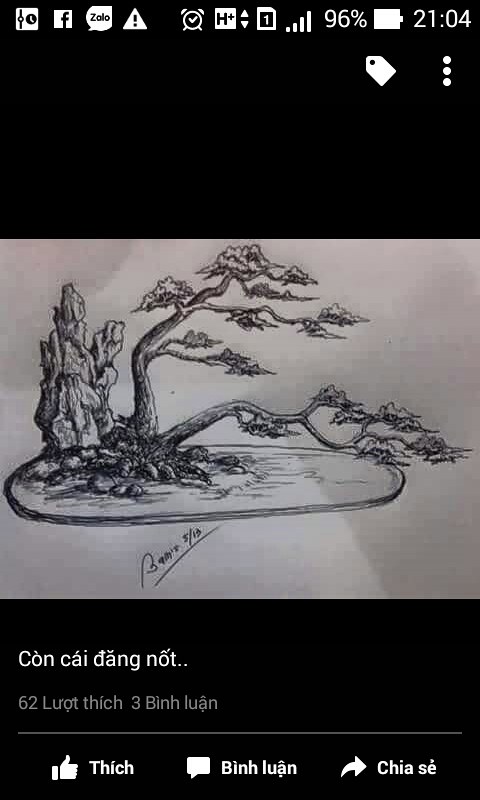This image is a screenshot taken from a smartphone displaying a Facebook post. The screen is predominantly black at the top and bottom, with the center featuring a gray rectangle containing a black-and-white drawing of a bonsai tree. The bonsai grows from a left-leaning trunk that splits into two branches, each adorned with foliage resembling cloud clusters. To the left of the trunk is an upright, jagged stone formation. The base of the bonsai and stone is an oval with intricate lining and shading. Text, seemingly in Vietnamese, is positioned below the drawing. At the bottom of the screen, there are three familiar icons: a thumbs-up like button on the left, a speech bubble comment button in the middle, and a share arrow on the right. The upper edge of the screenshot shows typical smartphone status icons, including app notifications, battery percentage, and the current time.